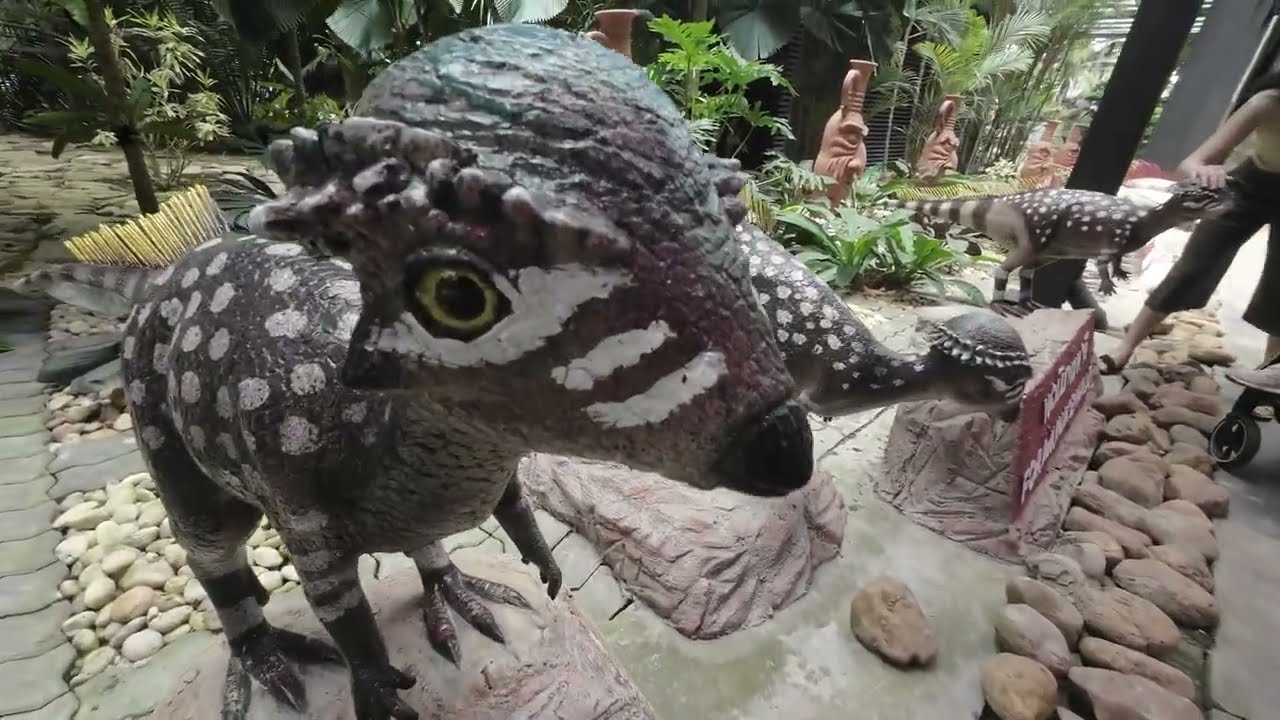The image showcases a detailed indoor display of lifelike ceramic or stone dinosaur models, intricately painted and posed to resemble real creatures. The focal point is a gray dinosaur with white polka dots on its back, white stripes on its face and limbs, standing upright on its hind legs, and featuring three-pronged bird-like claws. It has a distinguishable large yellow eye, a black beaky nose, and bony plates extending over its eyebrows and around its head.

Surrounding this central dinosaur are two more similarly designed models, each positioned in different poses to create a dynamic scene. A closer inspection reveals multiple rows of rocks and stepping stones leading into lush tropical greenery, enhancing the naturalistic setting. In the background, large pottery statues with face carvings add to the mystique of the exhibit.

Prominently, a person, partially visible, is bending down and petting one of the dinosaur models, adding a human element to the scene. Adjacent to this figure, there appears to be the wheel of a stroller with a child’s foot peeking out, suggesting a family-friendly environment. A sign with white text on a red background, though only partially visible, hints at providing further information about the display.